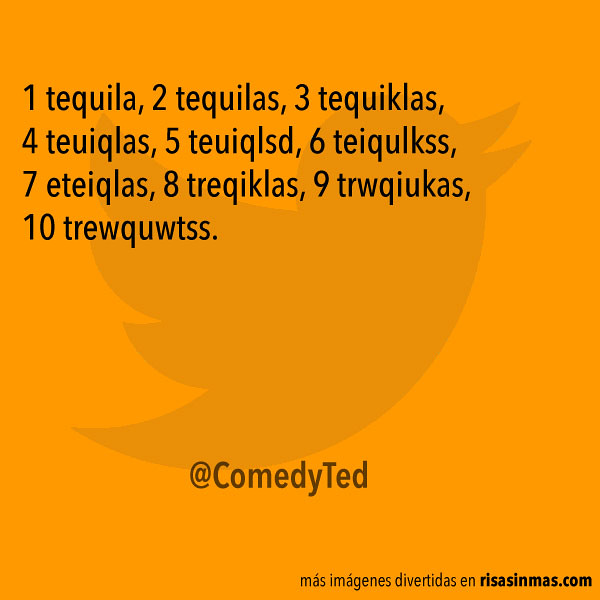The image depicts a vibrant orange square sign featuring a comedic theme. Dominating the composition is a large Twitter bird emblem situated centrally with a slightly darker shade of orange surrounding it. The main text humorously illustrates the progressive difficulty in spelling the word "tequila" as more drinks are consumed: "One tequila, two tequilas, three tequiklas," continuing until "ten," with increasingly jumbled letters. At the top left corner, the text begins clearly with "One tequila, two tequilas," and by the bottom, it devolves into a chaotic mix of letters. Below the Twitter bird, in prominent black lettering, it reads "@ComedyTed," emphasizing comedic content. In the bottom right corner, a bold website URL, "risasinmas.com," is displayed, alluding to more humorous images in Spanish.